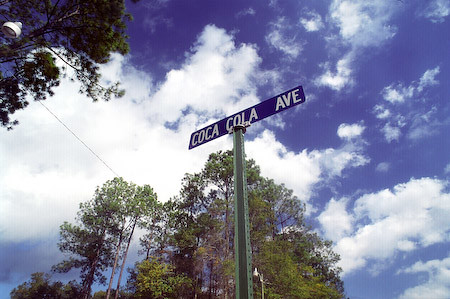The image showcases a street sign labeled "Coca-Cola Avenue" in bold white letters on a wide, blue rectangular background. The sign is mounted on a green metal pole, oriented diagonally from the bottom left to the top right. The scene is viewed slightly from below, highlighting the vivid blue sky adorned with large, white clouds predominantly occupying the left side of the frame. Tall, green trees with slim trunks are visible below the sign, extending towards the upper portions of the image. Additionally, several streetlights and power lines are positioned on the left side, adding depth and context to the urban setting.